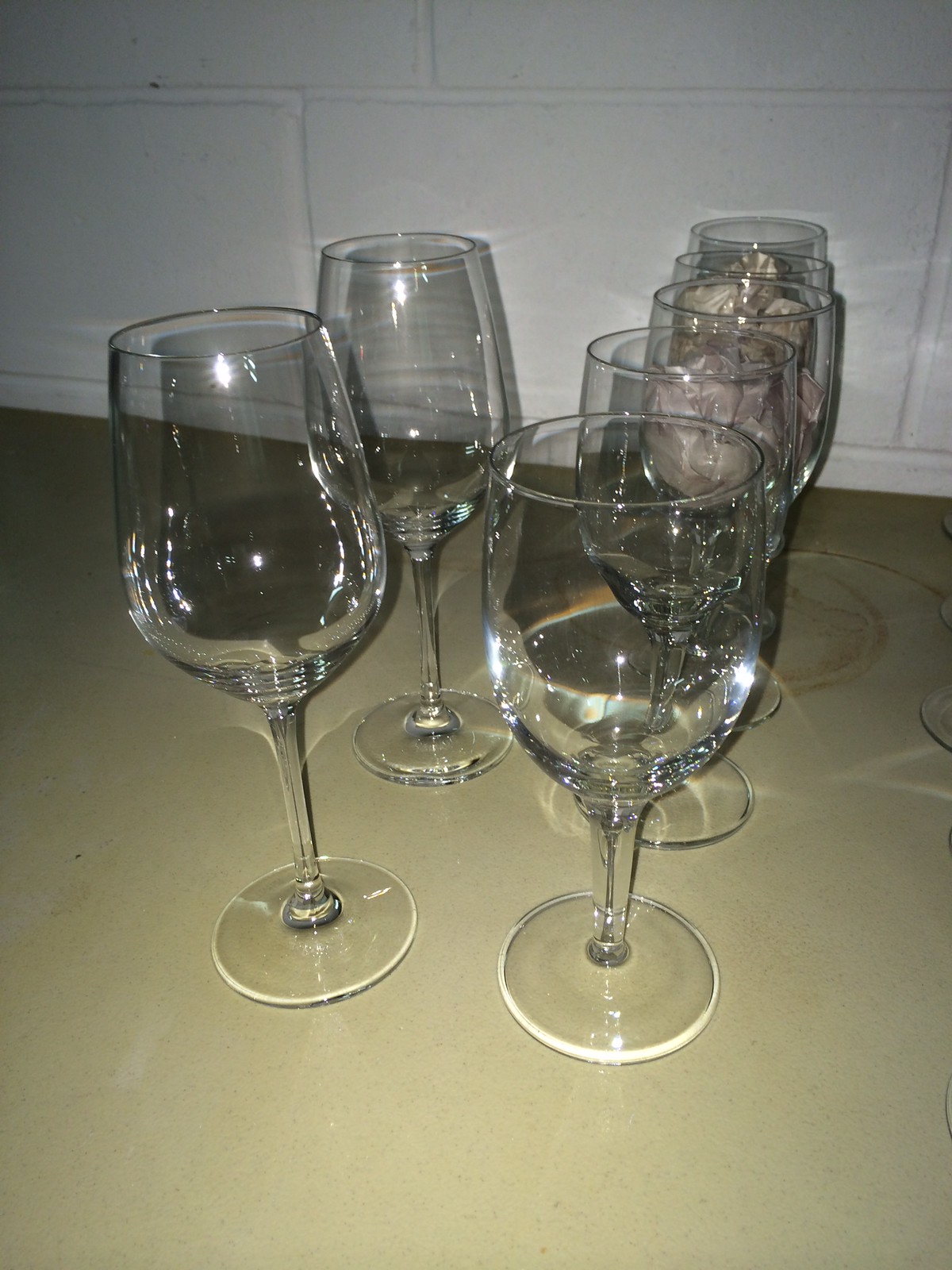The image is a photograph featuring an array of stemware glasses, typically used for wine, displayed on a glossy, light mustard-colored countertop, which has an old, Formica-like appearance. This surface showcases a noticeable browned ring stain in the back right, presumably left by a hot pot or pan. The backdrop consists of a white-painted breeze block wall with clearly visible mortar lines, equally painted in white.

In the arrangement, there are seven wine glasses of slightly varying shapes and sizes. On the right side, five glasses are lined up in a row receding from the camera's perspective. Of these, the front two are empty, while one in the middle contains a crumpled object—potentially paper or fabric. On the left side of the image, two glasses stand separately; these appear to be taller and made of smoky gray transparent glass. The glasses all have round bottoms, narrow necks that widen towards the bowl, and their surfaces reflect light, creating various highlights and illuminated spots across the scene.